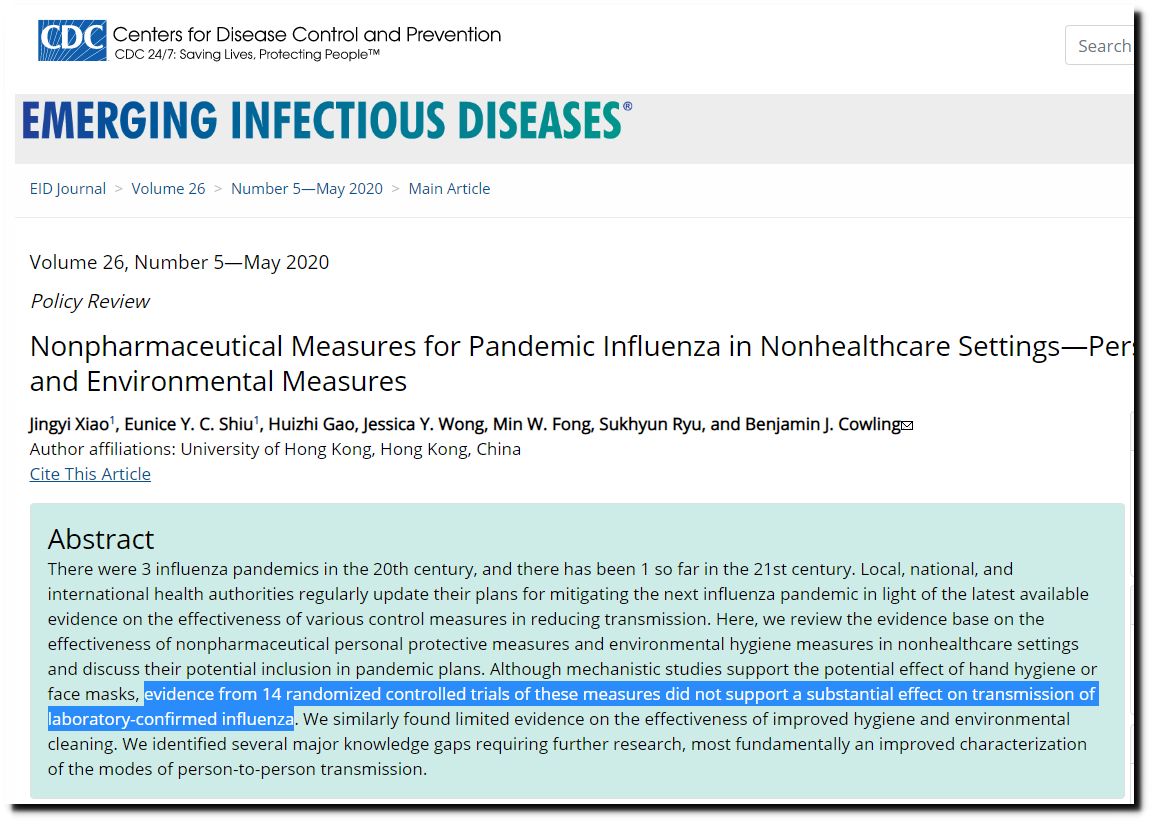Screenshot from the CDC's Website on Emerging Infectious Diseases

In the upper left corner, the screenshot prominently features the CDC logo, a blue rectangle with "CDC" in bold, white letters. To the right of the logo, the full name "Centers for Disease Control and Prevention" is displayed. Beneath this, the tagline "CDC 24/7: Saving Lives, Protecting People" appears in smaller font. In the top-right corner of the screenshot, there is a search bar for navigating the CDC website.

Below the CDC logo, the title "Emerging Infectious Diseases" is prominently displayed in bold, capital letters. This particular page is from Volume 26, Number 5, dated May 2020. Below the date, it is indicated that the content is a policy review article titled "Non-Pharmaceutical Measures for Pandemic Influenza in Non-Healthcare Settings: Personal and Environmental Measures."

The article's authors are listed next, with a total of seven names. Most of the authors are affiliated with the University of Hong Kong, Hong Kong, China.

Beneath the list of authors, a greenish box contains the article's abstract. Highlighted in blue within this box are the significant findings: "Evidence from 14 randomized controlled trials of these measures did not support a substantial effect on transmission of laboratory-confirmed influenza."